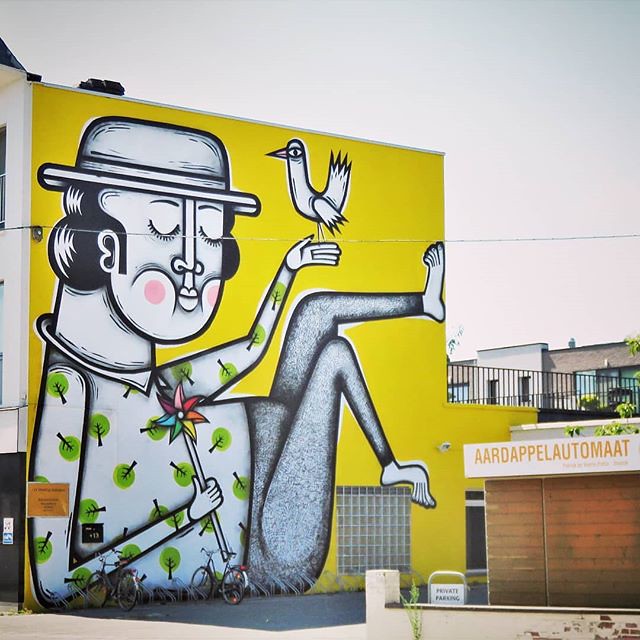The image showcases a large, yellow mural painted on the side of a building, depicting a reclining caricature of a person with black hair, dressed in a white shirt adorned with green tree patterns and trousers, but no shoes. The person's eyes are closed, cheeks flushed, and they are sporting a white horn-like hat. They hold a bed in their left hand and a pinwheel in their right, with a bird perched above their left hand. The figure’s right foot rests on a window on the building's wall, and their left foot is positioned above this window, reaching towards the wall's edge. At the base of this mural, two bicycles are parked. The wall also features black railings at the top. In the far background, there is a house, while closer to the viewer, there is a smaller building with the name "A-A-R-D-A-P-P-E-L Automat" written across it, visible on the opposite side of the street.